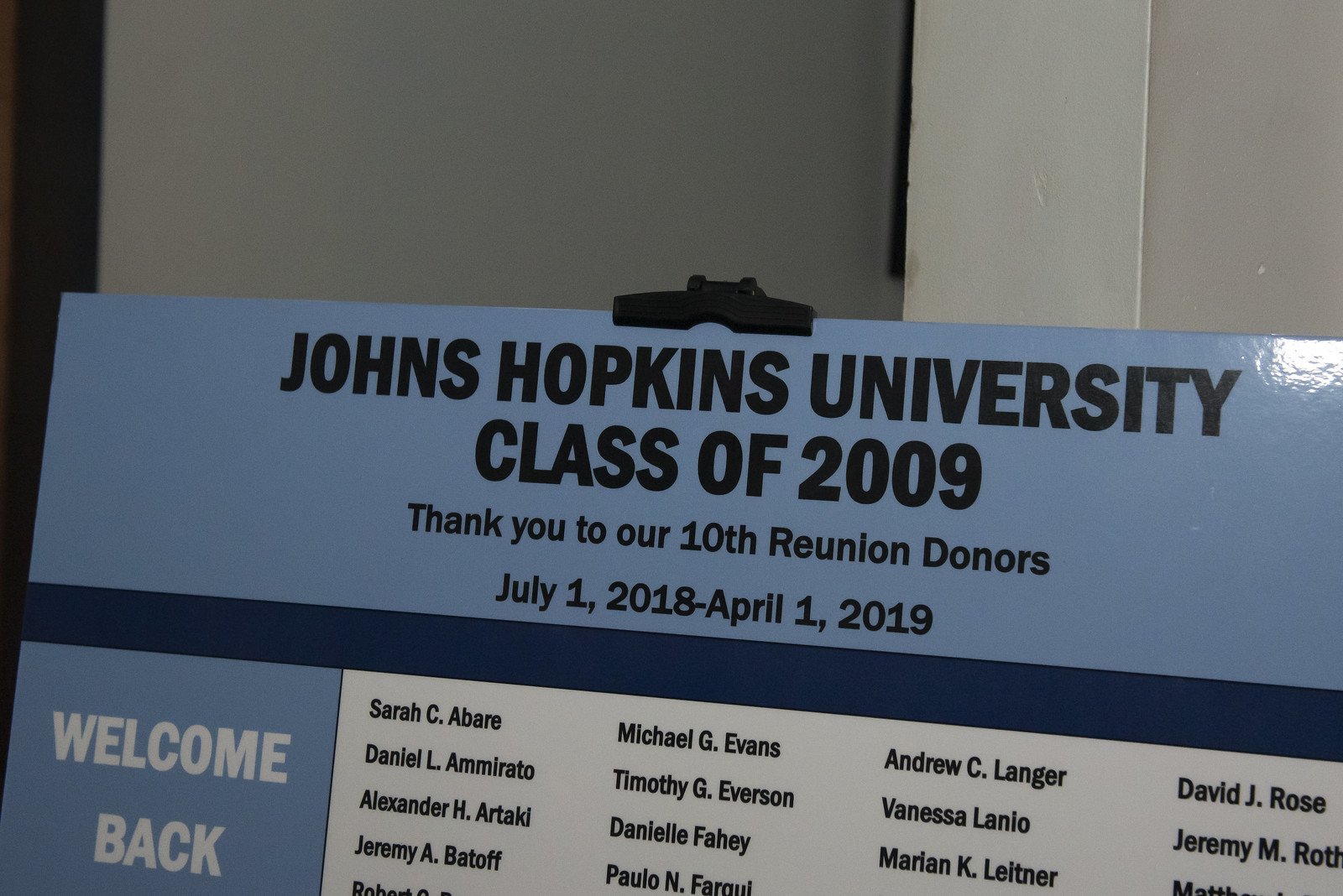The image depicts a donor recognition display for Johns Hopkins University's Class of 2009. The display, set indoors, showcases a light baby blue rectangular sign at the top, featuring black text that reads: "Johns Hopkins University Class of 2009. Thank you to our 10th reunion donors. July 1st, 2018 to April 1st, 2019." Beneath this, on the lower left-hand side, there's white text saying "Welcome back." Below the introductory text, the display transitions into a large white section listing the names of donors: Sarah C. Avery, Daniel L. Amato, Alexander H. Artaki, Jeremy A. Botoff, Michael G. Evans, Timothy G. Everson, Daniel Valle, Paolo N. Faraghi, Andrew C. Langer, Vanessa Lino, Marion K. Leitner, David J. Rose, and Jeremy E. M. Roth. At the bottom of the image, the view cuts off some of the text, leaving parts of the names like "Matthew" partially visible and incomplete. The entire display is framed against a background with blue, dark blue, white, and red hues, capturing a daytime indoor setting within a collegiate environment.